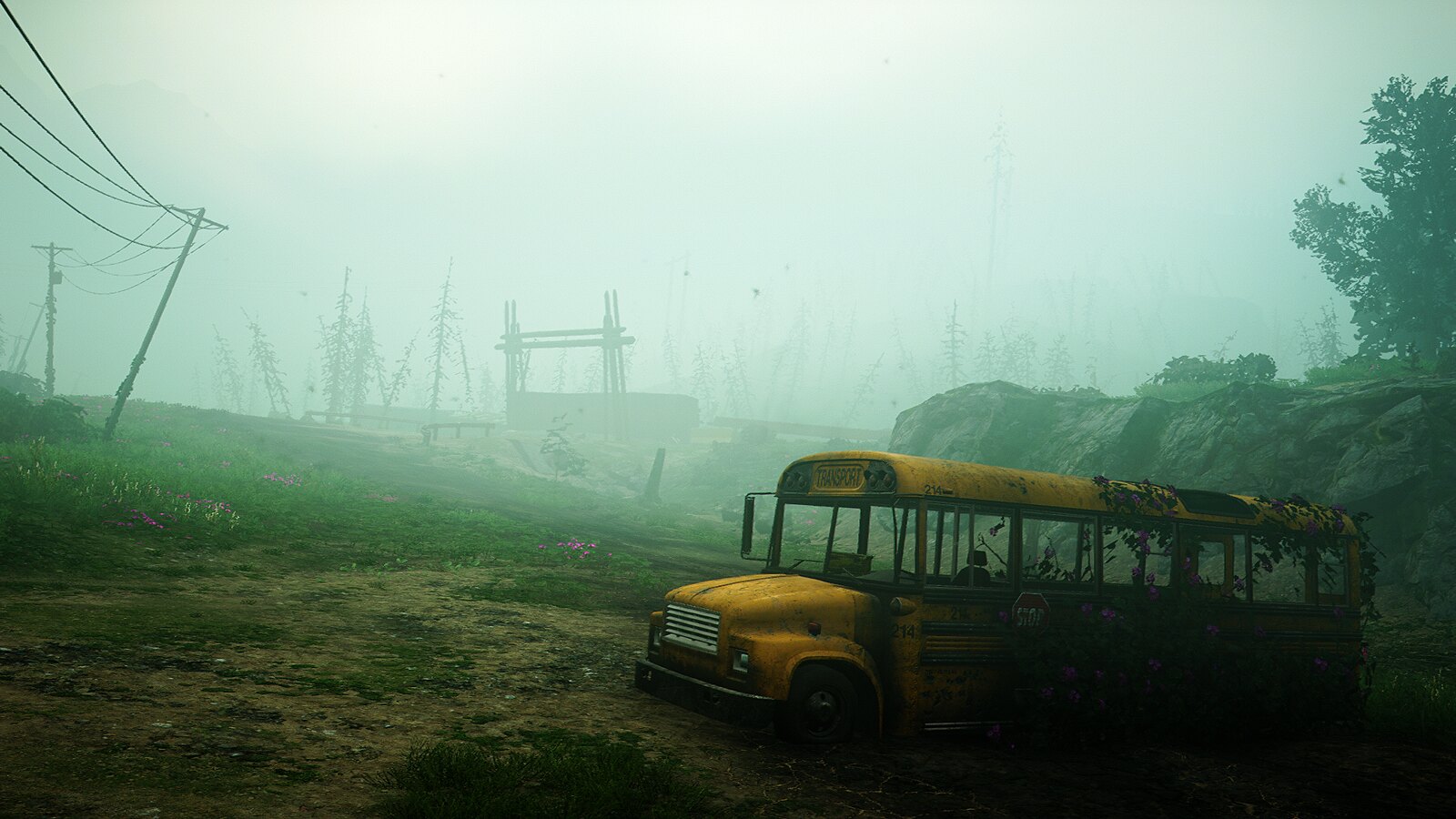This color image, likely a screenshot from a video game, depicts a decaying, post-apocalyptic landscape cloaked in a hazy, greenish fog, evoking a sense of desolation. In the lower right corner, a weathered yellow school bus with a prominently protruding nose is gradually being reclaimed by nature, with ivy creeping up from the mid-section towards the back and covering the windows. The bus, which bears the classic "school bus" marking with black stripes and two rear windows, appears abandoned and forgotten.

Dominating the upper right section of the image are several rough-looking utility poles, with one particularly jagged pole leaning noticeably to the right, in stark contrast to its adjacent upright counterparts. The wires extend upwards and towards the left, adding to the chaotic ambiance.

The background reveals dead, spindly trees and a large wooden structure, possibly a bridge, with upright and horizontal beams forming a T-shape. This structure spans above a valley-like depression, framed by a rock wall stretching from just right of center to the far right side of the scene. The rocky outcrop has a deciduous tree or bush perched atop it, suggesting a struggle for survival in this barren environment.

The ground in the foreground is a mix of patchy brown dirt and scattered green weeds and grass. The sky overhead is ominously gray and hazy, further contributing to the eerie, end-of-the-world atmosphere that pervades this desolate wasteland.